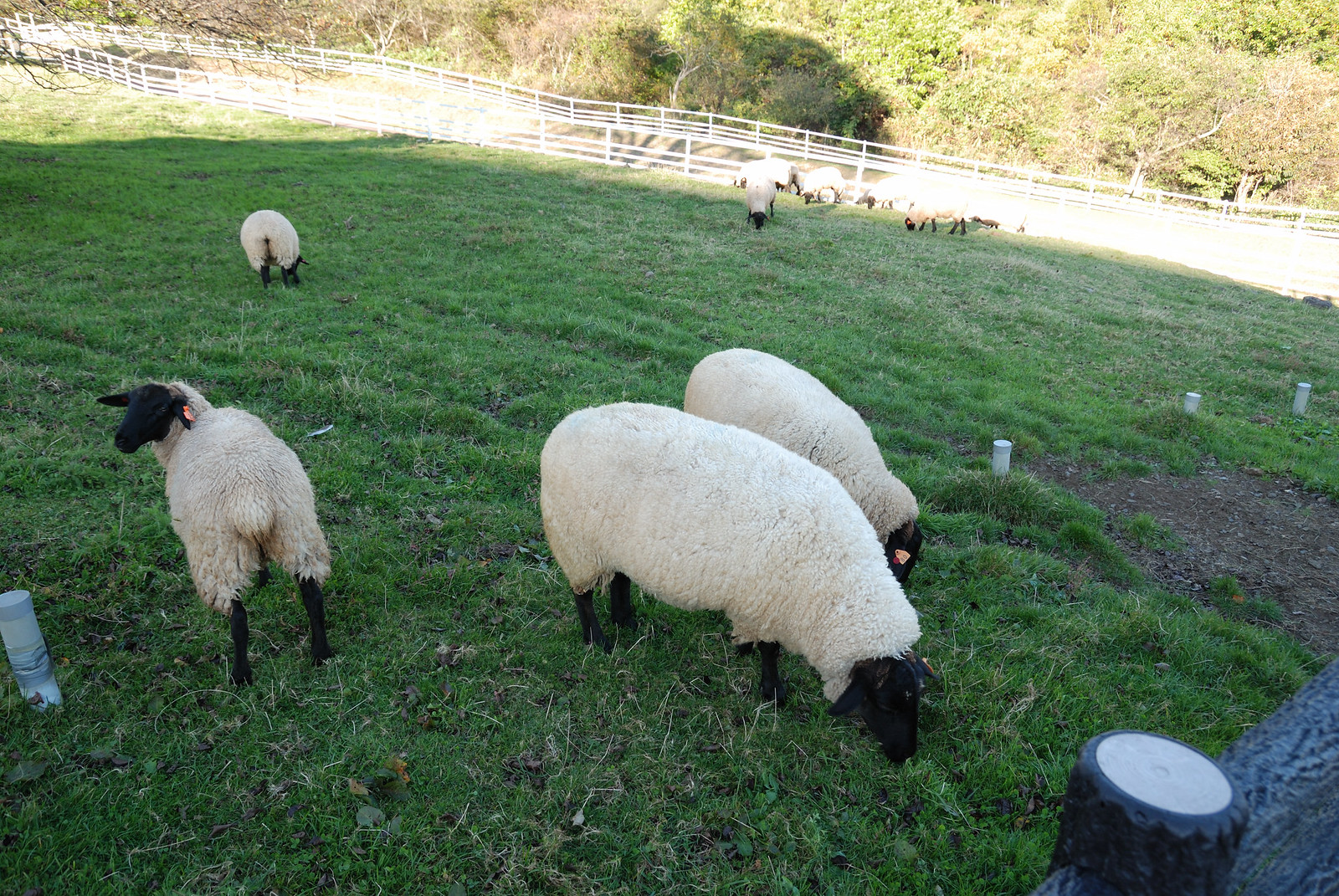In this photograph, a lush green pasture is depicted, enclosed by a white timber fence running from the top left to the right side of the image. In the foreground, there are three main sheep: two, at the center, are engrossed in munching on the short green grass, and one, slightly to the left, looks back over its shoulder. These sheep are mostly off-white with thick woolly coats, contrasting with their black faces and legs. Ear tags, most likely pink, are visible, providing a hint of farm management. 

Adding to the scene, a wooden fence segment is visible in the bottom right corner, serving as a juxtaposition to the white fence. Towards the top left, partially concealed by the grazing sheep, another sheep's hindquarters can be spotted, while several more sheep cluster in the sunlit background, appearing less distinct due to the light. 

Beyond the fenced area lies a dense forest, casting shadows over parts of the field. Three white PVC pipes with caps protrude from the ground on the right side, hinting at some form of infrastructure. The overall atmosphere suggests a tranquil, well-maintained farm or ranch, on a late spring or early summer day.